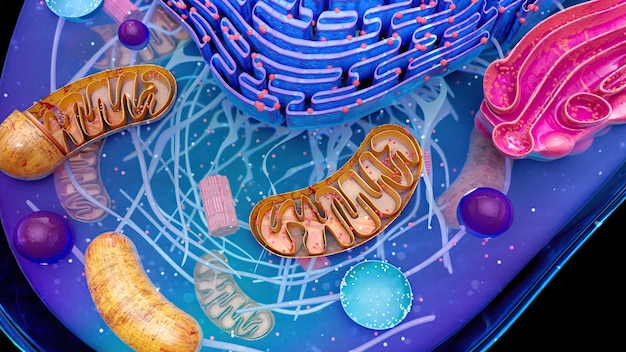This image is a detailed and colorful artistic mock-up of a cell featuring various organelles and structures in a vibrant palette. The primary background is dark purple, setting off an intricate depiction of cell components. The main features include three kidney bean-like structures, likely representing mitochondria, in light orange. One of these mitochondria is fully intact, another is cut in half, and the third has a smooth portion on the left side with a cross-sectional view on the right, revealing internal pathways or formations. In the upper right quadrant, there's a bright pink area adorned with vessels and cup-like structures. At the center of the cell, a blue maze-like network with red dots and light blue lines captures attention. Additionally, various colorful globes are scattered throughout: a blue circle with white dots, a purple circle outlined in blue, and a pink oblong feature. These elements, some shown in cross-section, contribute to the detailed and intricate portrayal of cellular anatomy.